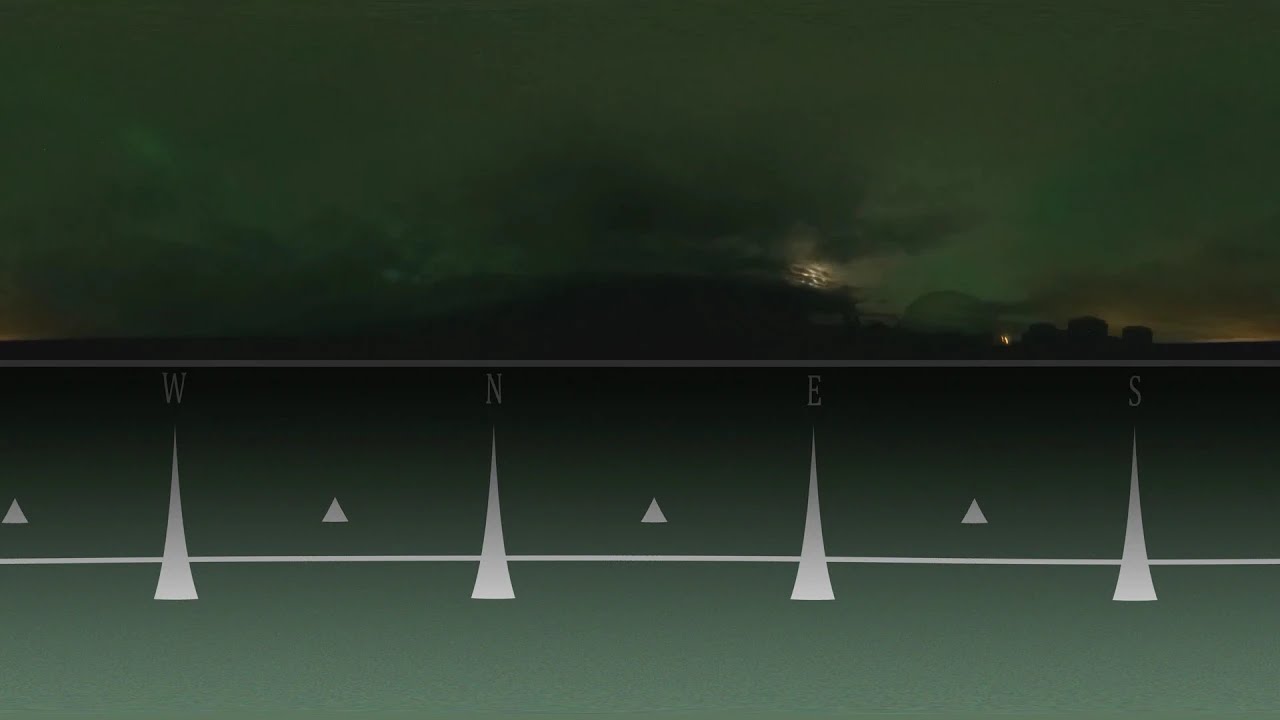The image depicts a mysterious and eerie outdoor scene dominated by a dark green background. Thin horizontal white lines cut across the image, with the one near the bottom running the entire width and another slightly above it, darker in shade, doing the same. At the center, there is a prominent triangle, surrounded by arrows from a compass pointing towards the letters W, N, E, and S, each followed by a smaller triangle. The letter W is slightly darker than the others.

A dark green skyline of mountains stands in the background. On the right side, there are a couple of very dark-colored trees, next to a small orange light. Just to the left of the center, a faint light shines through, hinting at either a hidden moon or some light source akin to a sunset, as indicated by a splash of yellow color at the edge of the horizon.

The overall atmosphere is foggy and smoky, with an unsettling blend of dark green and occasional orange hues, creating a sense of a surreal, almost horror-like setting. There are no people present, and the vague outlines of buildings suggest a haunted, desolate place you would dread to find yourself alone in. The strange compass and the monochromatic palette add to the unsettling ambiguity of the scene, making it look like something out of a nightmarish vision.